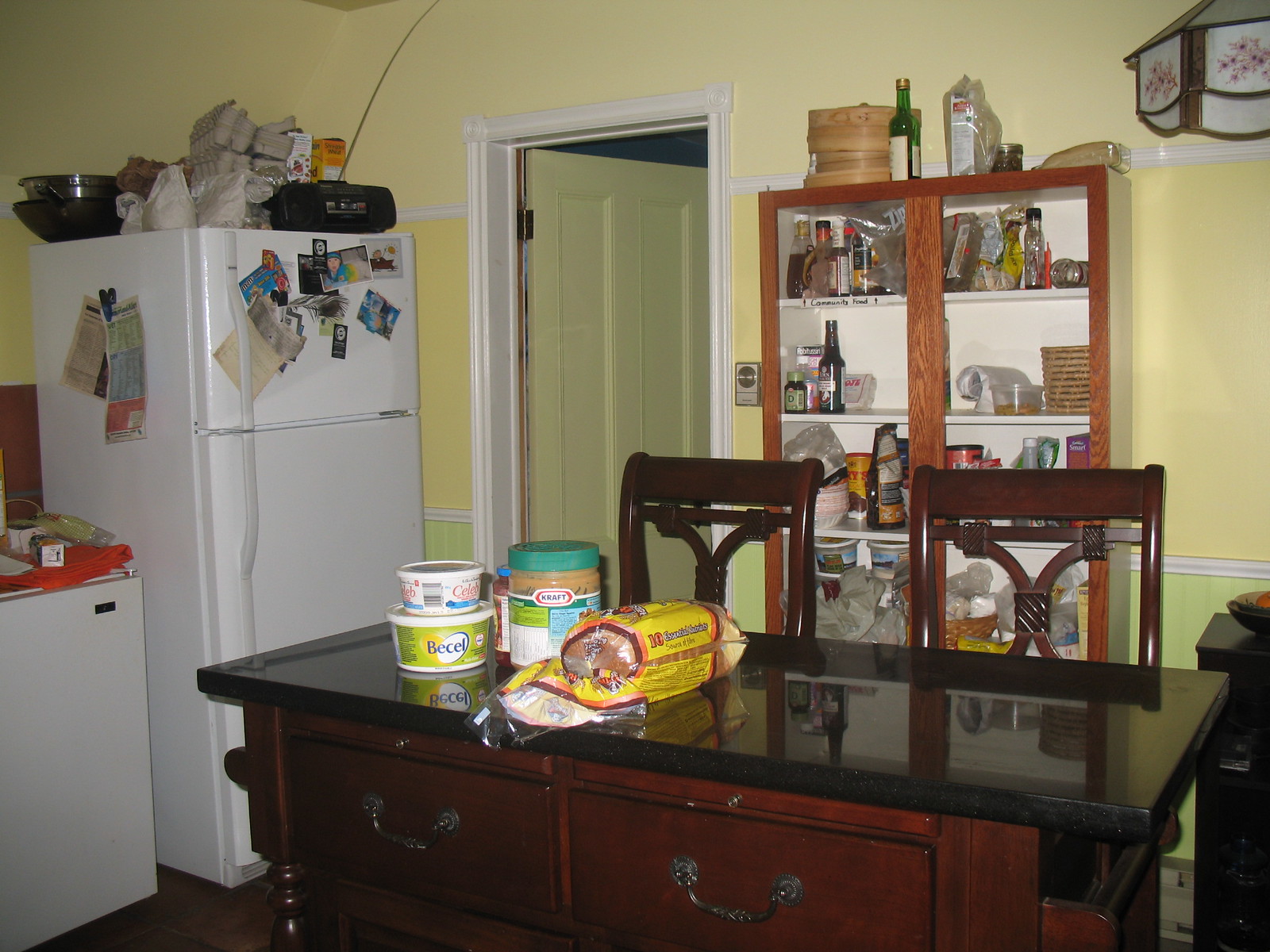The image depicts a kitchen with distinctive features and various items. The background showcases yellow walls that morph into a greenish hue towards the bottom, separated by a white trim. Central to the image is an open doorway which reveals a yellowish-white door ajar behind it. To the right, there's a pantry cabinet stocked with an array of food items, and it houses bottles of wine or other liquids—one on top and one inside.

On the left side of the image stands a two-part white refrigerator adorned with numerous magnets and a variety of items such as boxes and egg crates on top, along with a black radio. Adjacent to the fridge is a smaller white mini-fridge, topped with an orange item.

Dominating the center of the room is a dark brownish-red bar table accompanied by two matching bar stools positioned behind it. Alongside the table, a black countertop is visible, holding a loaf of bread, a brown jar of peanut butter with a blue lid, a green container with a white lid, and another white container with a white lid.